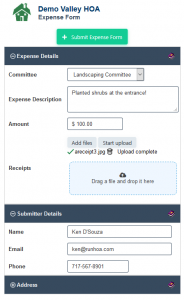The image appears to be a screenshot of an expense form from a homeowners association website, specifically for "Demo Valley HOA." The interface, mostly white and formatted for mobile viewing, features a simplistic layout and various form fields.

At the top, there is an icon of a single-story house with a green roof and chimney, followed by the text "Demo Valley HOA" in blue. Below this header, in black, is the title "Expense Form." 

Centrally located is a prominent green button with a plus sign, labeled "Submit Expense Form." Beneath this button is a blue horizontal bar spanning the width of the screen, containing a circular icon on the left and the text "Expense Details." Adjacent to this, on the right, is a blurry pinkish icon.

In the "Expense Details" section, a white box appears, labeled "Committee," and inside it, "Landscaping Committee" seems to be selected. Another box follows, titled "Expense Description," where the description reads "Planted Shrubs at the Entrance" and the amount is "$100."

Two smaller boxes are located below for file management: "Add Files" on the left and "Start Upload" on the right. There is a small green arrow beside a message indicating that a JPEG file named something like "Receipt 3" has been successfully uploaded, marked as "Upload Complete."

On the left side, the text "Receipts" is visible, while a blue box on the right suggests dragging and dropping files with the instruction "Drag a File and Drop it Here."

Further down, another blue bar is present, this time labeled "Subscriber Details," with similar circular and pink icons. This section includes fields for "Name," "Email," and "Phone Number," filled with the details: "Ken Osuza" (slightly blurry), "ken@notsure.com," and "717-66x-8901," respectively.

Lastly, there is a blue bar for "Address," again featuring the circular and pinky-purple icons, although the address details are not clearly visible in the image.